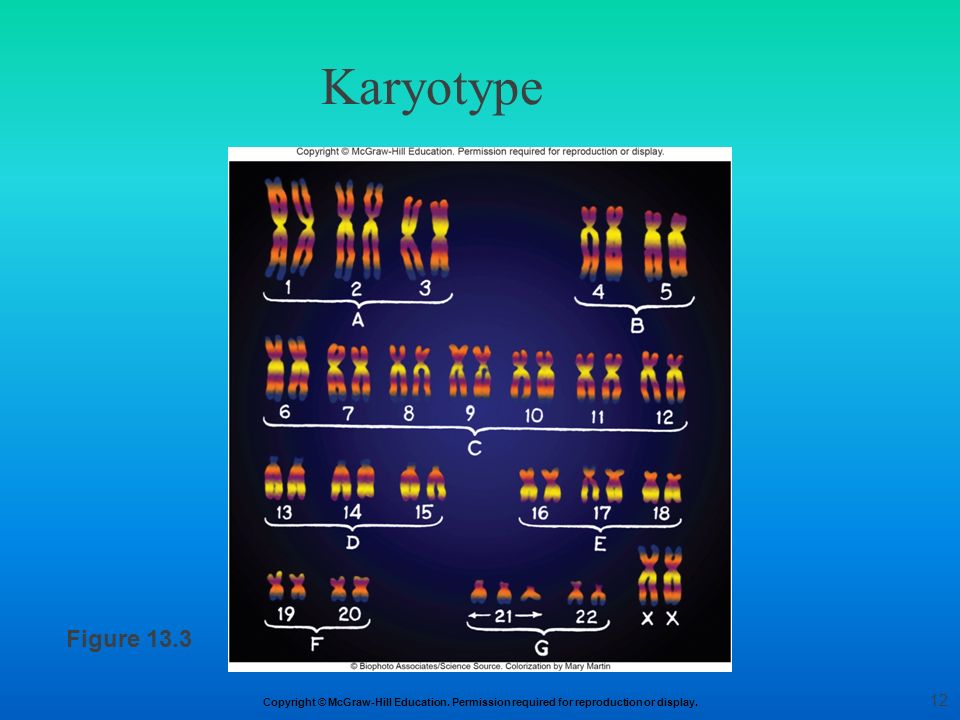The image illustrates a karyotype diagram with a comprehensive depiction of chromosomes against a light blue background. Titled "Karyotype," it bears the copyright notice "Copyright by McGraw-Hill Education, Permission Required for Reproduction or Display" both at the top and bottom. The diagram is labeled as Figure 13.3 and features distinct sets of chromosomes arranged in pairs, color-coded in a rainbow sequence—blue, orange, purple, yellow, and blue—starting from the center and extending to the tips.

Set A contains three of the largest chromosome pairs labeled 1, 2, and 3. Set B, slightly smaller, comprises pairs 4 and 5. Set C includes the next range of pairs, labeled 6 through 12. Set D has three pairs, numbered 13 through 15, while Set E also comprises three pairs labeled 16 through 18. Set F contains two pairs, 19 and 20, and Set G includes the last two pairs, 21 and 22. Additionally, in the bottom right corner, there are two X chromosomes labeled XX, completing the karyotype presentation.